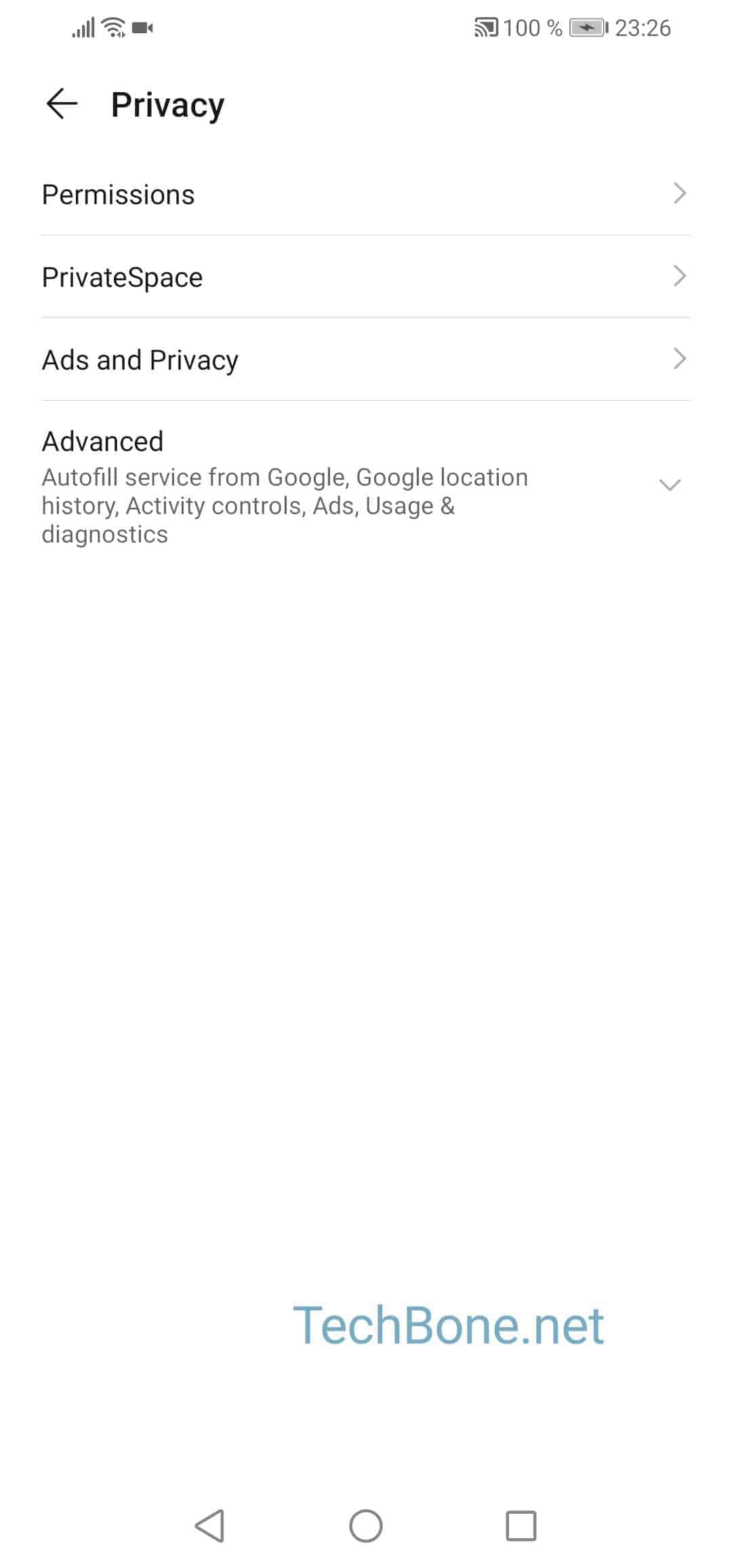The image displays a cell phone screen with detailed interface elements. At the top of the screen, the status bar shows full Wi-Fi signal strength and a 100% battery level. The current time is indicated as 23:26. Below the status bar, a series of menu items are listed. The first line is highlighted in bold black text and slightly larger than the rest, featuring a left-pointing arrow followed by the word "Privacy." Subsequent lines list various menu options: "Permissions," "Private Space," "Ads and Privacy," and "Advanced." Additional items under the "Advanced" category include "Auto Fill Service from Google," "Google Location History," "Activity Controls," "Ads," and "Usage and Diagnosis." At the bottom of the screen, the words "TECHBONE.NET" are prominently displayed in larger, blue, capitalized letters.